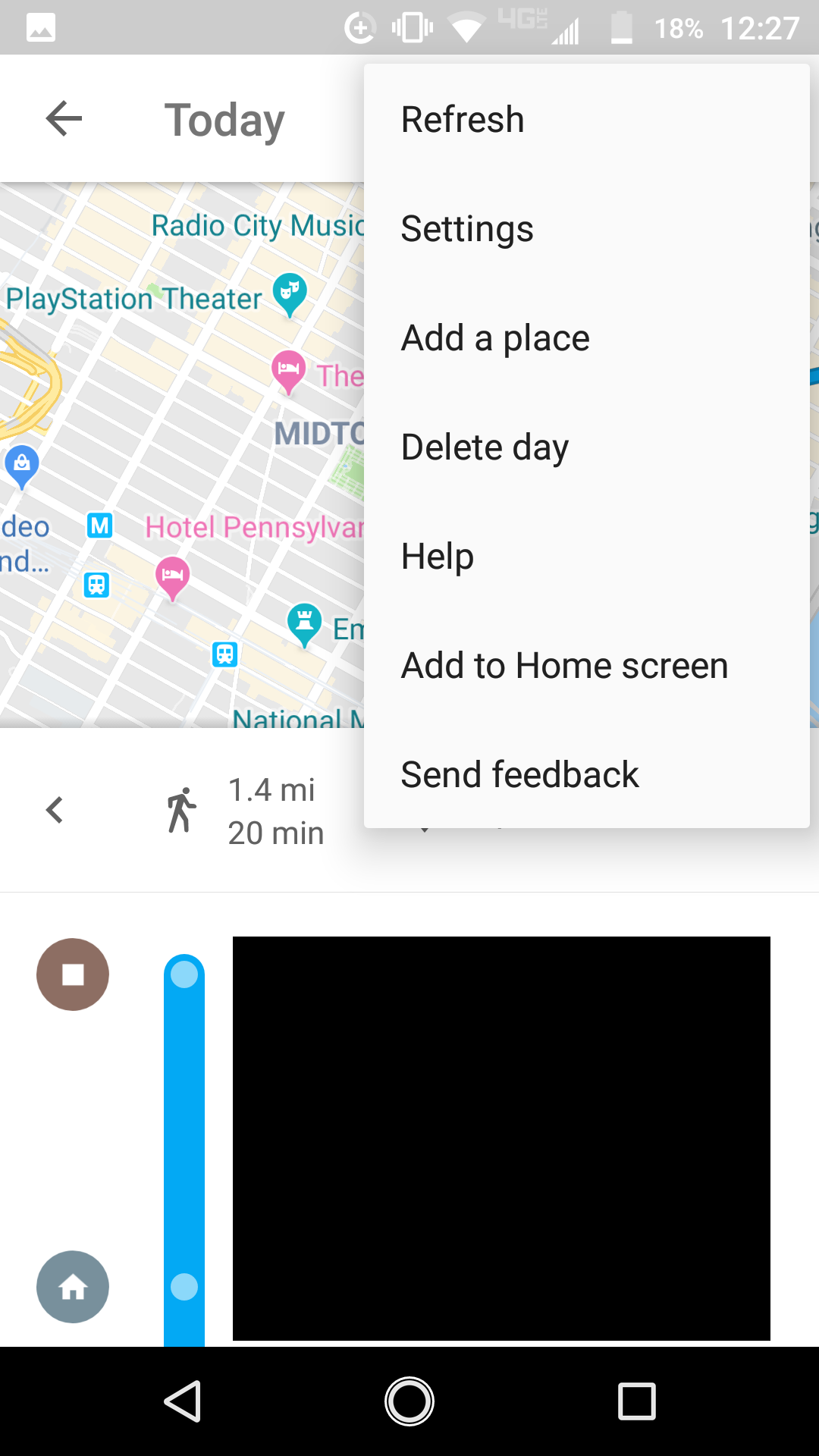A detailed caption for the screenshot provided:

"This screenshot captures the complete display of a navigation app on a smartphone. The background is predominantly white. At the very top, a gray horizontal status bar is visible, showcasing various icons starting from the left. There is an icon indicating that a screenshot was recently taken, followed by a plus sign, a vibrate icon, a Wi-Fi symbol showing three out of four bars, a 4G LTE signal icon, and a cell signal icon with five bars denoting full reception. The battery level is shown to be 18%, and the time displayed is 12:27.

The main content of the screen is a map highlighting a location near Radio City Music Hall, Hotel Pennsylvania, and PlayStation Theater. The menu within the navigation app is open, revealing several options listed in black: refresh, settings, add a place, delete day, help, add to home screen, and send feedback.

At the top of the map, a route is displayed with navigation details showing a distance of 1.4 miles and an estimated walking time of 20 minutes. Additionally, there is a black square at the bottom of the screen, presumably covering sensitive information."